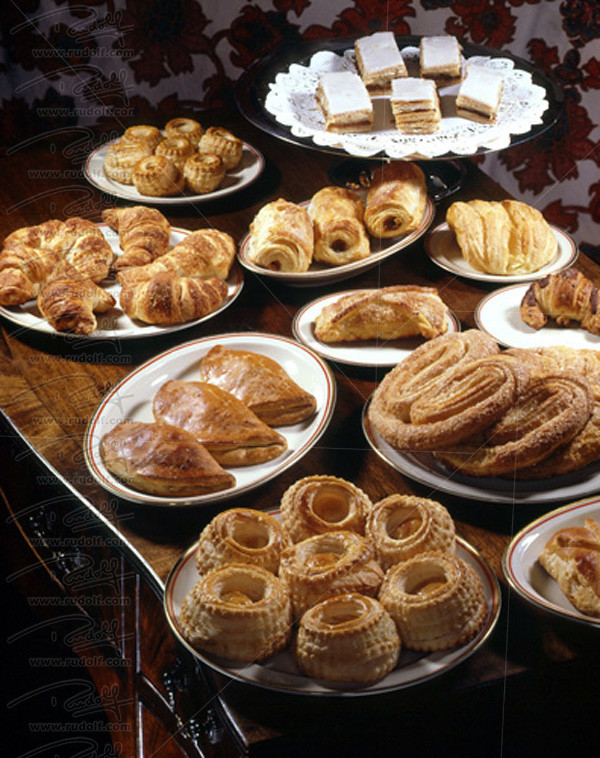The image captures a meticulously arranged assortment of pastries and desserts on a large, vintage-looking brown wooden table. Various white plates with elegant red and gold rims hold an array of baked goods, including curved croissants, turnovers, pretzels, tiramisu, cannolis, and other enticing pastries. A distinctive black circular plate, slightly elevated on a stand, showcases rectangular desserts with white frosting and layered fillings atop a lacy white doily. The surrounding plates display a visually appealing mix of crispy, browned pastries, some with powdered sugar or frostings. The background features a wallpaper with large reddish floral designs on a white backdrop, adding a charming, old-fashioned ambiance to the scene. The wooden floor underneath the table further enhances the rustic aesthetic. A translucent watermark with a repeated signature logo and the website URL www.rudolph.com runs along the left border of the image. This picturesque setting exudes a cozy, inviting atmosphere, reminiscent of scenes found in cookbooks or culinary blogs.